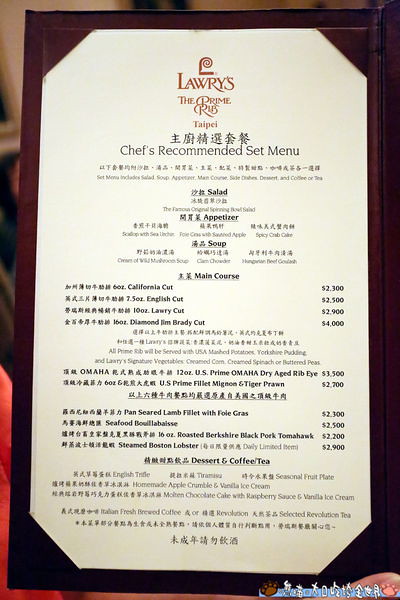This photograph showcases a menu encased in a sleek black vinyl cover with a transparent plastic sheet overlaying printed paper. At the top, an elegant red letter "L" introduces the restaurant name "Lawry's" followed by the phrase "The Prime Rib" and the location "Taipei," all in red lettering.

The majority of the text is in black and interspersed with Asian characters. Below the header, the menu announces a "Chef's Recommended Set Menu." Unfortunately, the following two lines are not legible. 

Further down, the menu itemizes:
- **Salad**, followed by two unreadable lines.
- **Appetizer**.

Next, it lists:
- **Soup**, with the specific details unreadable.
- **Main Course**, featuring entries like:
  - California Cut priced tentatively at $2,300.
  - 7.5 oz English Cut at $2,500.
  - A 10 oz Lawry Cut at $2,900.
  - Diamond Jim Brady Cut at $4,000.
  - An Omaha 12 oz U.S. Prime Omaha Cut.

The menu continues with around six more standard menu lines that are not legible. At the end, it highlights a section for **Dessert and Coffee/Tea**. 

Each English menu item is preceded by Asian script, indicating the multicultural presentation of this upscale dining experience.